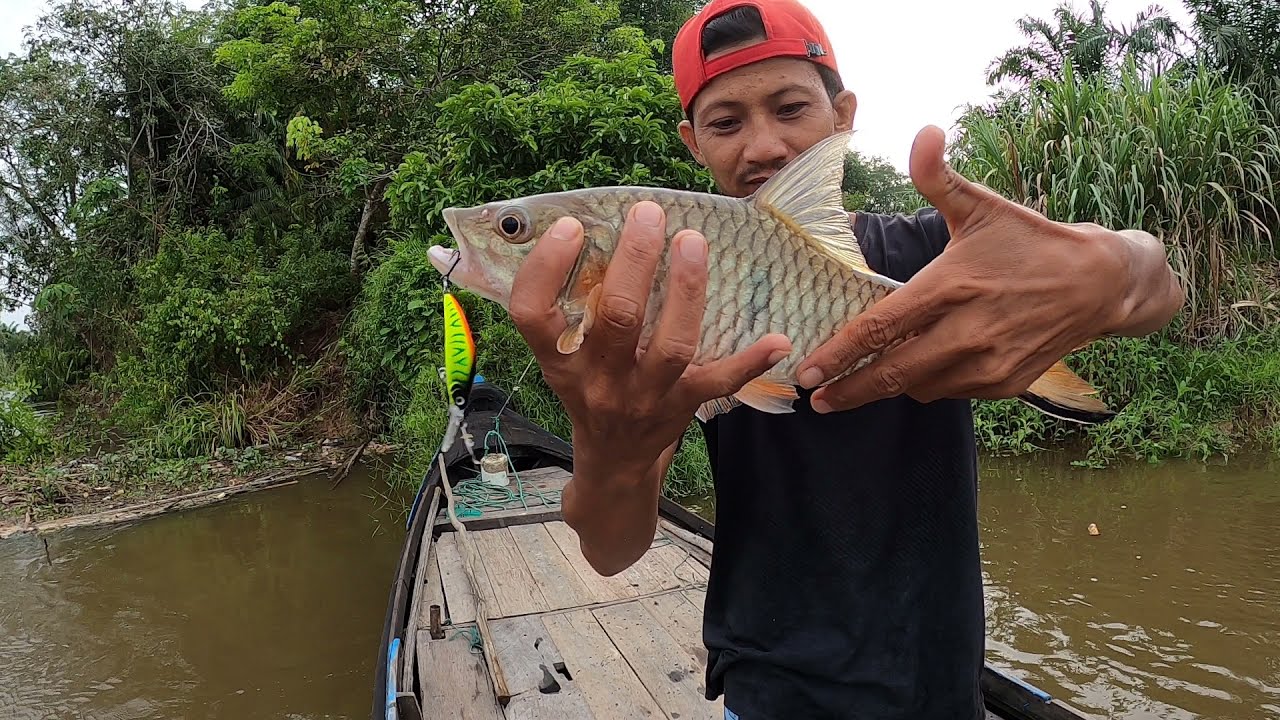In this detailed image, a man of likely Asian descent stands in a small, old wooden boat close to the muddy shoreline. Wearing a backward orange baseball cap and a short-sleeved black t-shirt, he uses both hands to proudly hold up a recently caught fish with a hook still in its mouth. The fish is of a decent size, with a lighter coloration of white and orange. The muddy water beneath the boat is brown, creating a stark contrast with the varied shades of green from the trees and plants that populate the background. The setting appears to be an outdoor, midday scene, with a glimpse of light blue sky visible above the trees. The focus remains on the man and his catch, as he gazes at the fish rather than the camera, amidst an array of natural colors including tan, light brown, light green, and red, adding depth and texture to the photograph.